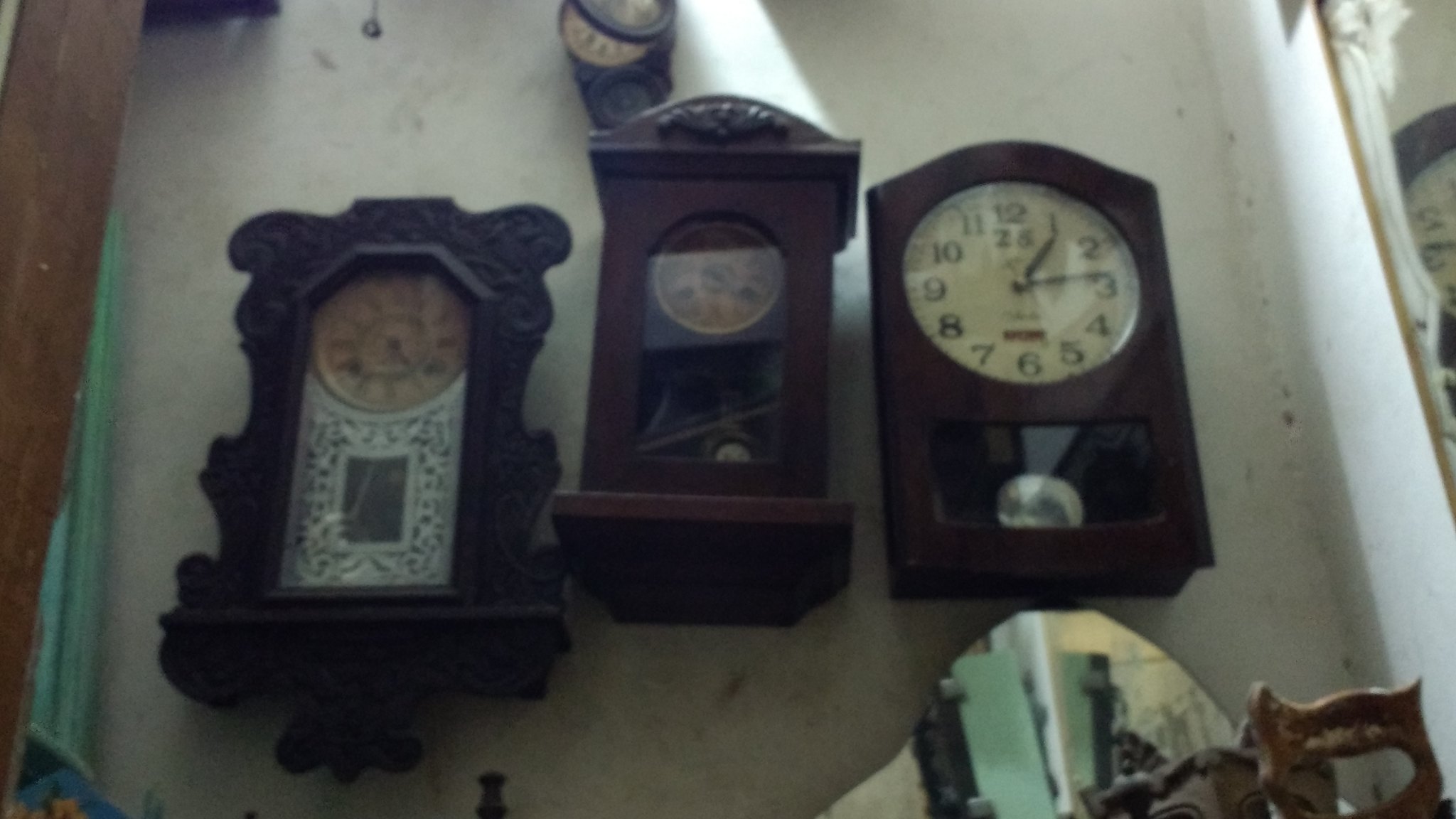The photograph depicts three antique-style wall clocks, each encased in dark wooden housings, reminiscent of miniature grandfather clocks with visible pendulum mechanisms. The clocks are arranged together against what appears to be an old and dirty wall, although another perspective suggests they might be laid flat on a wooden floor with the picture taken from above. The clock faces have aged over time, with two showing a noticeable brown tint on what was once white. Each clock displays a different time, hinting that they may no longer be functional.

The leftmost clock features an intricate metal grill decoration in front of its mechanism and a detailed wooden frame, adorned with Roman numerals on its face. The middle clock is smaller with a notably tiny clockface. The right clock has the largest dial, displaying bold, black numerals. A handsaw’s blade is partly visible at the lower right corner of the image, adding to the vintage ambiance and cluttered setting of the photograph.